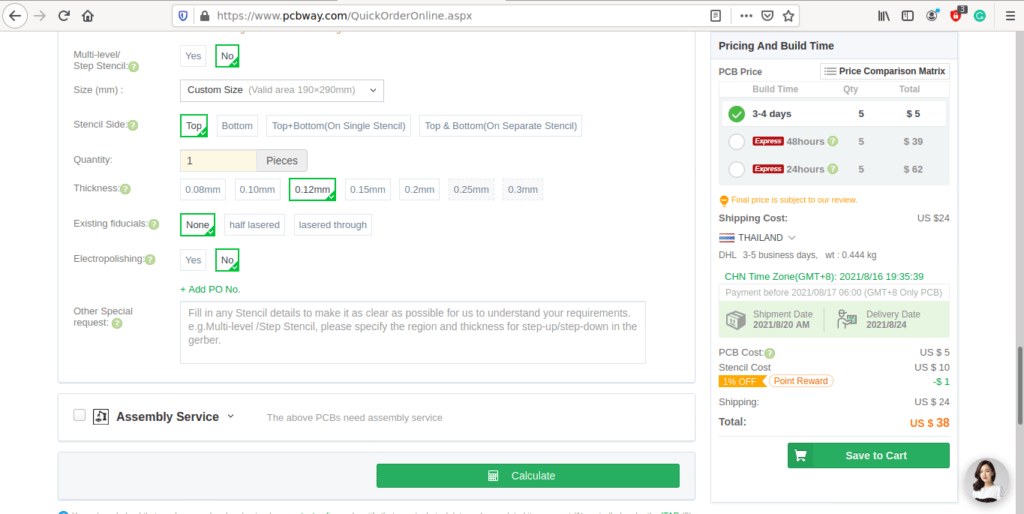**Screenshot of Web Page for PCB Stencil Order on PCBWay**

The image is a detailed screenshot of a web page from the URL "www.pcbway.com/quick_order_online.aspx". At the top of the screenshot, the address bar is visible, showcasing the website's address. To the right of the address bar, there are some logos along with an icon of three lines indicating a drop-down menu.

Below the address bar, a selection form for ordering a multi-level step stencil is presented. The form fields and their current selections are as follows:

1. **Stencil Type**:
   - Multi-Level Step Stencil (Selected option: No)

2. **Size in Millimeters**:
   - A drop-down menu for custom size selection with a valid area range of 190 to 290 millimeters.

3. **Stencil Position**:
   - Options available are Top, Bottom, and Top plus Bottom (Selected option: Top).

4. **Quantity**:
   - Pieces: 1

5. **Thickness Options**:
   - 0.08 mm
   - 0.1 mm
   - 0.12 mm (Selected)
   - 0.15 mm
   - 0.2 mm
   - 0.25 mm
   - 0.3 mm

6. **Existing Fiducials**:
   - None (Selected)
   - Half-Lasered
   - Lasered Through

7. **Electro Polishing**:
   - Yes
   - No (Selected)

8. **Other Special Requests**:
   - There is a text input field with a placeholder text that reads: "Fill in any stencil details to make it as clear as possible for us to understand your requirements. EJ, multi-level, step stencil, please specify the region and thickness for your step-up, step-down in the Gerber."

This comprehensive display exemplifies the interface for customizing and ordering a stencil from PCBWay, detailing the various parameters and options available for precision tailoring to specific manufacturing needs.